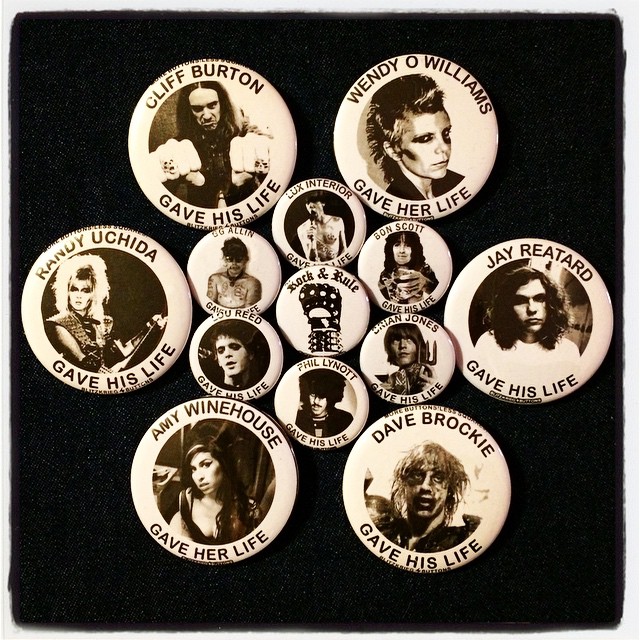The image depicts a black piece of felt fabric adorned with a collection of buttons featuring deceased musicians. Arranged in a structured pattern, there is a central small button featuring a fist clad in a spiked leather glove with the phrase "Rock and Rule" inscribed above it in a medieval font. Surrounding this central button are six larger buttons, each approximately 1.5 inches in diameter, and an additional six smaller buttons, around 1 inch in size, forming a concentric circle.

Each button showcases a black and white photograph of a musician, with their name arched above the image and the words "gave his life" or "gave her life" below, indicating their dedication and ultimate sacrifice for the craft of music. The identified musicians include Cliff Burton (Metallica), Wendy O. Williams, Jay Reatard, Dave Brockie, Amy Winehouse, Randy Uchida, Gigi Allen, Lux Interior (The Cramps), Bon Scott (AC/DC), Lou Reed (The Velvet Underground), Brian Jones (The Rolling Stones), and Phil Lynott (Thin Lizzy). This poignant collection symbolizes a tribute to the musicians' enduring influence and the legacy they left behind.